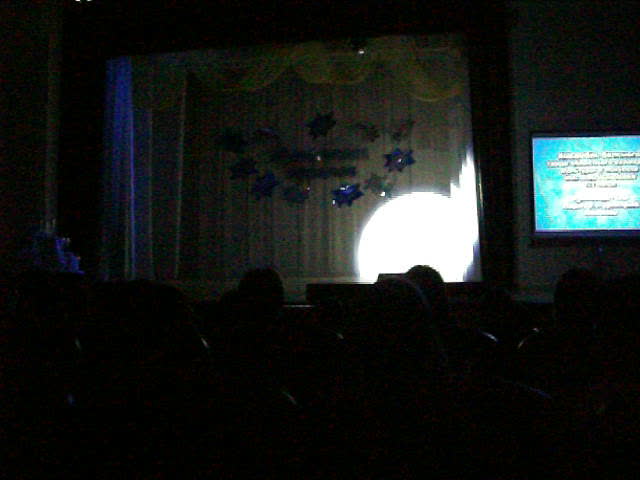The image depicts a dark theater setting, taken from the audience's perspective. In the foreground, the silhouettes of several rows of people's heads are visible, emphasizing the view of someone seated among the audience. The stage ahead is dimly lit, with a prominent spotlight shining in its bottom right corner. The backdrop of the stage features a curtain adorned with blue and silver foil stars encircling some text that's difficult to decipher. To the right side of the stage, an LCD monitor displays text on a blue background, possibly providing information related to the upcoming performance or presentation, although the words themselves are unreadable due to blurriness.